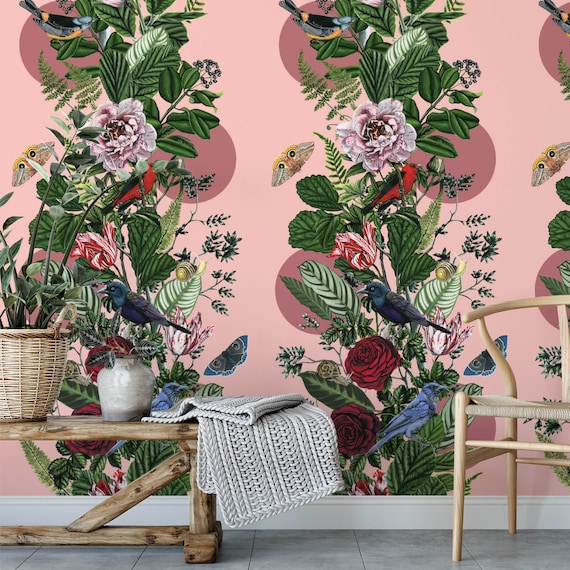The image displays a vibrant scene characterized by a bold and colorful wallpaper that adorns a pink wall with white baseboard trim. The wallpaper features a repeating pattern every few feet, reinforcing its decorative nature. Intricate designs boast tropical foliage, red roses, pink peonies, and carnations intertwined with an assortment of birds, including blue and orange birds, red cardinals, and a blackbird. Yellow and blue butterflies add to the lively aesthetic.

In the foreground, a rustic bentwood armchair with a rope seat sits to the right, while a low wooden bench made of logs and featuring a triangular post against a straight leg occupies the left. The bench is topped with a gray and white striped folded rug, a woven wicker basket brimming with greenery and flowers, and a ceramic vase with additional blooms. The setting rests on a gray tiled floor, emphasizing a blend of natural textures and vibrant, decorative details.